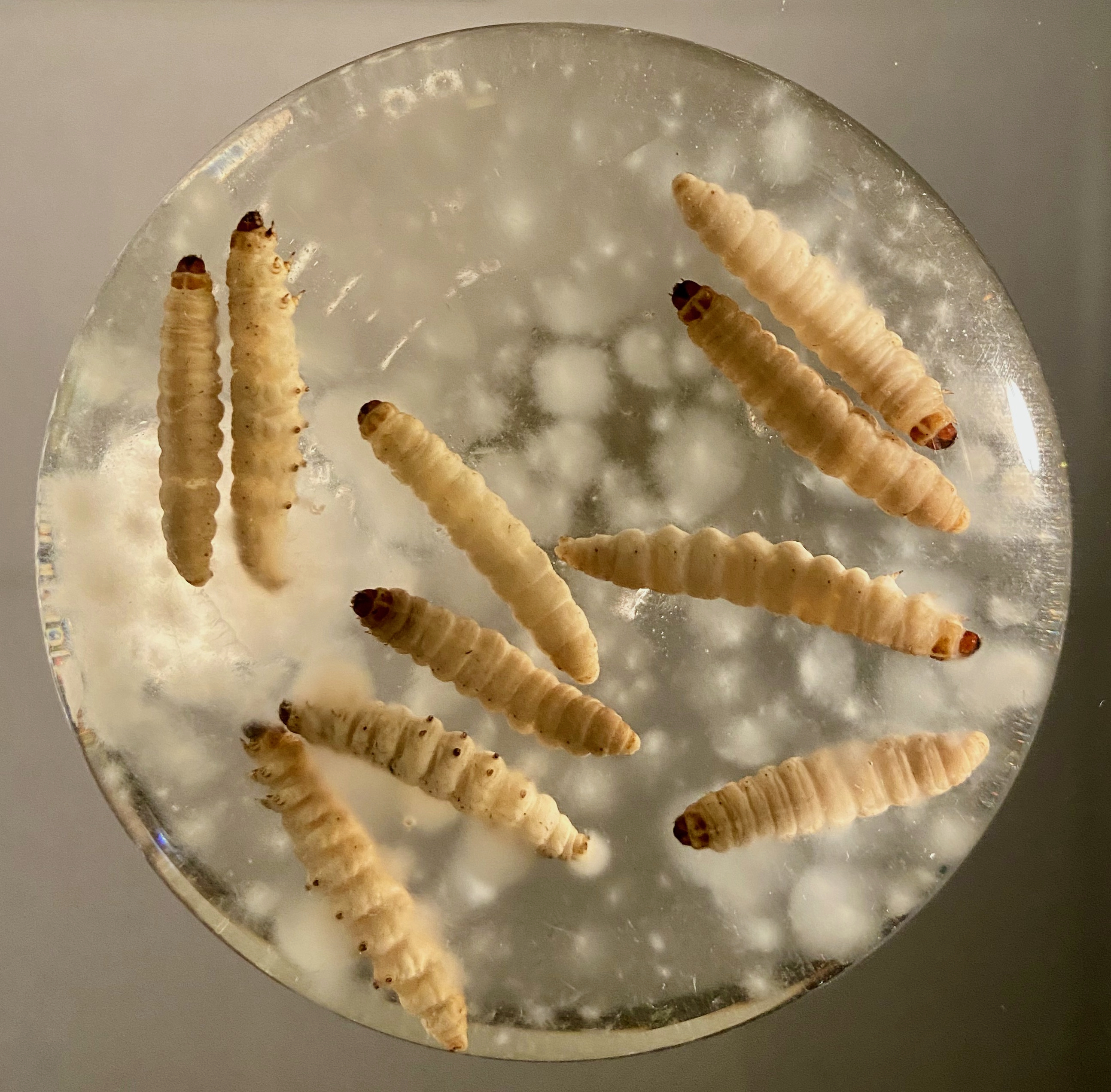The image features a close-up of several maggots or caterpillar-like insects encased within a translucent, spherical object that could be made of glass, resin, or possibly ice. The sphere, which forms the central focus of the picture, shows a range of transparency, with sections appearing cloudy. The insects inside are beige or tan in color, each with a dark brown or black head and tiny legs that are visible on some of them. The background transitions from a light gray to a darker gray, providing a stark contrast to the clear yet somewhat clouded sphere. The textured bodies of the maggots, with their ridged backs, are arranged at different angles inside the sphere, adding to the detailed, almost scientific or artistic nature of the image. Despite its intriguing composition, the image may evoke a sense of discomfort due to the close-up view of the insects.